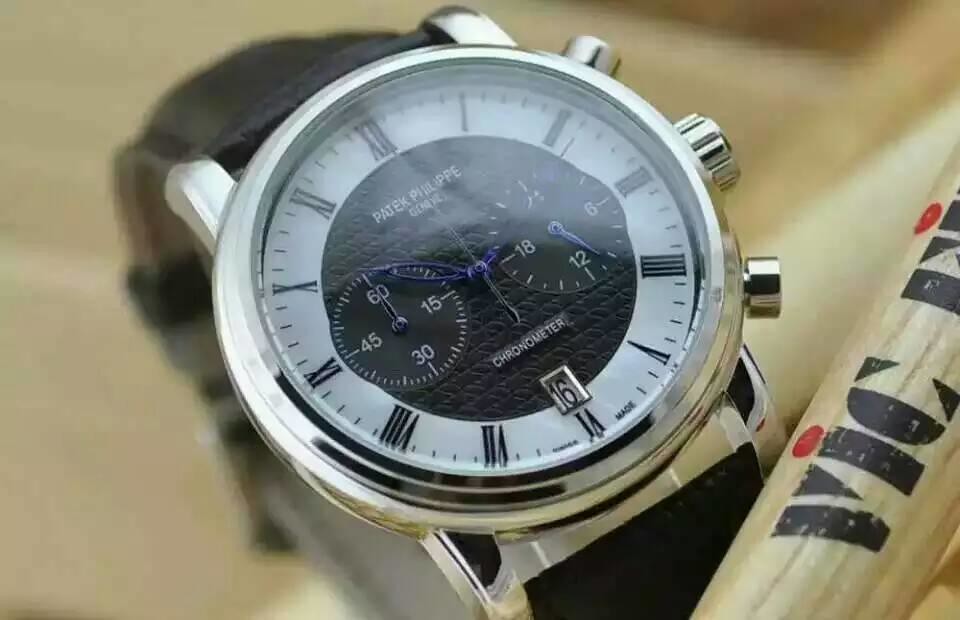This indoor color photograph provides a detailed close-up view of a sophisticated Patek Philippe wristwatch, showcasing its intricate design and functionalities. The shot captures the watch face tilted slightly to the left, with the 12 o'clock position pointing to the upper left corner and the 6 o'clock position pointing to the right. The watch features a silver body with a round face, highlighting an elegant contrast between its black center and a white outer ring where the black Roman numerals are displayed.

At the center of the watch face are two smaller sub-dials; the one on the left appears to display seconds, marked with numbers from 0 to 60, and the one on the right potentially shows hours, marked with numbers from 0 to 24. The hands of the watch and those of the sub-dials are black, giving it a refined look. Above the center, under the 12 o'clock position, the brand name "Patek Philippe" is inscribed in white lettering on the black background. Just below the center, the word "Chronometer" is elegantly displayed in silver letters.

The watch also features a date complication, visible through a small silver rectangle just above the 6 o'clock position, displaying the number 16. The watch is equipped with three silver knobs on its right side, aiding in its various functions and time-setting mechanisms. The wristband is portrayed as being crafted from black leather, adding to its luxurious appeal.

In the background, a light tan hue dominates, intersected diagonally by what appears to be a round, light wooden stick, possibly a baseball bat, with the word "VIC" printed in black letters and a red dot accentuating the 'I'. The image is well-focused and brightly lit, enhancing every minute detail of the watch and its surroundings.